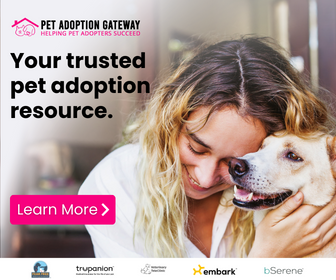Caption: 

"Introducing Pet Adoption Gateway – your trusted resource for successful pet adoptions. This informative graphic features a cozy image of a woman lovingly snuggling with a small dog, perfectly capturing the joy pets bring into our lives. The center of the design prominently showcases a logo with a small house, a puppy, and a cat, all set against a pink backdrop. Key messages like 'Helping Pet Adopters Succeed' are highlighted in pink, while 'Pet Adoption Gateway' and 'Your Trusted Pet Adoption Resource' are clearly displayed in black for easy readability. At the bottom, the credibility of the platform is emphasized with logos of five accredited services, ensuring users of the website's reliability and secure transaction processes. Dive in and learn more – because every pet adoption story deserves a happy beginning."